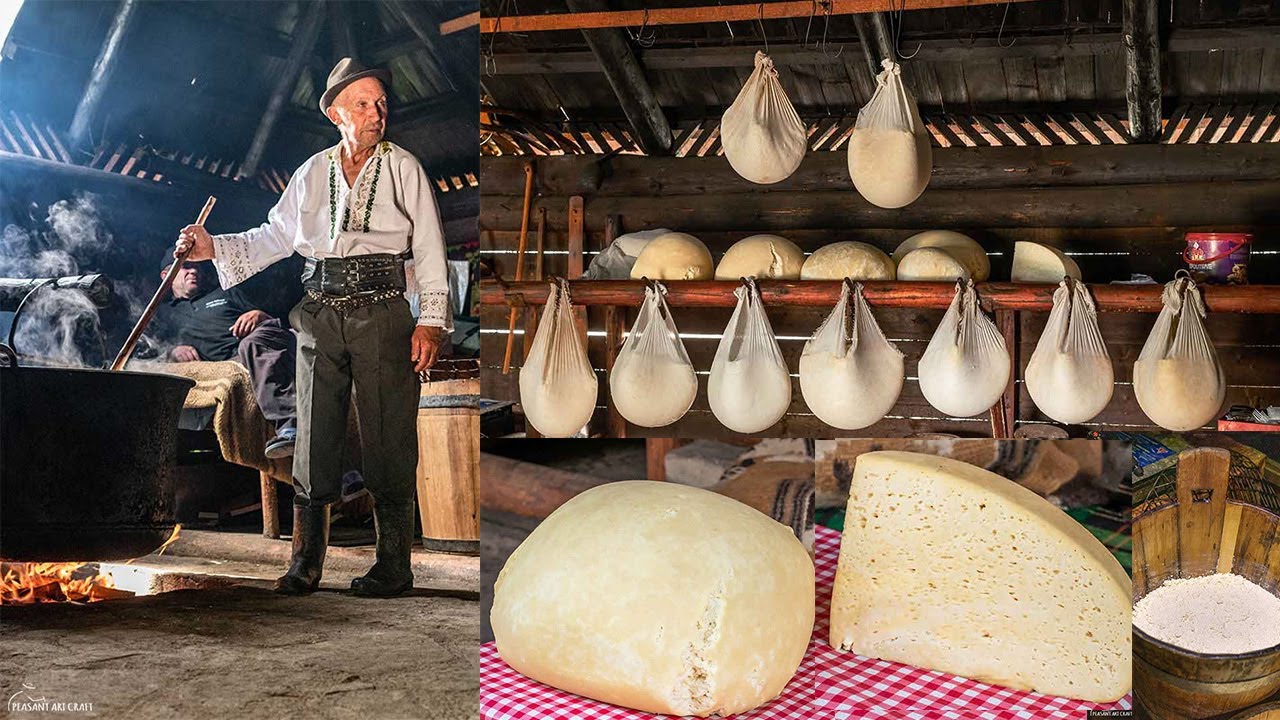The image portrays an older gentleman of lighter skin complexion, positioned on the left-hand side, dressed in traditional attire reminiscent of a German outfit. He wears a dark green hat matching his dark green pants, a white long-sleeved shirt tucked into his pants with a thick black belt, and dark brown high boots that resemble rain boots. The man is engaged in stirring a large black kettle using a long-handled spoon or rod, with visible fire underneath the pot, suggesting he is likely cooking or making cheese.

In the background on the right-hand side, there is a table draped with a red and white checkerboard tablecloth displaying large chunks of cheese, including what appears to be Swiss cheese and white cheese. Above and around the table, various sacks and bags are hung from wooden beams inside a barn-like setting, contributing to an old-fashioned, farmer's market ambiance. The scene is brightly lit with natural light, giving the image a clear and detailed appearance. The overall composition and attire of the man hint at a historical or cultural German context.